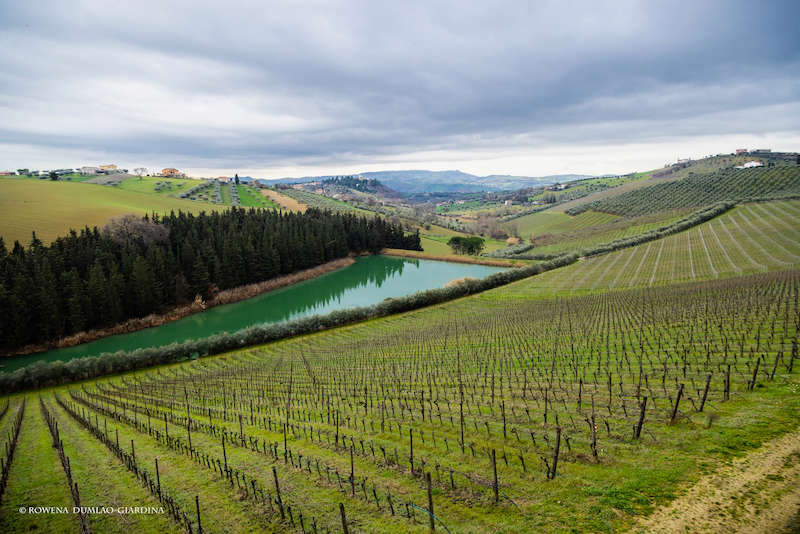The photograph captures a cloudy, daytime scene of a picturesque, hilly landscape viewed from atop a small hill. In the foreground, a grassy field slopes downward, peppered with rows upon rows of wooden stakes, likely used for growing crops. This field extends significantly to the right side of the image. Directly in front of the field is a triangular-shaped body of water with a greenish hue, possibly an irrigation canal. Beyond the water, a dense stand of evergreen trees forms a natural barrier leading to more expansive fields and meadows. To the far left and right, these fields stretch into the distance, dotted occasionally by bushes, additional trees, and various buildings. In the far background, the land rises into rolling hills and mountainous terrain. The sky occupies a quarter of the upper portion of the photo, filled with light gray and off-white clouds. Subtle details, including unreadable text at the bottom left and the varied shades of green, brown, and almost black, enhance the scene's complexity and depth.